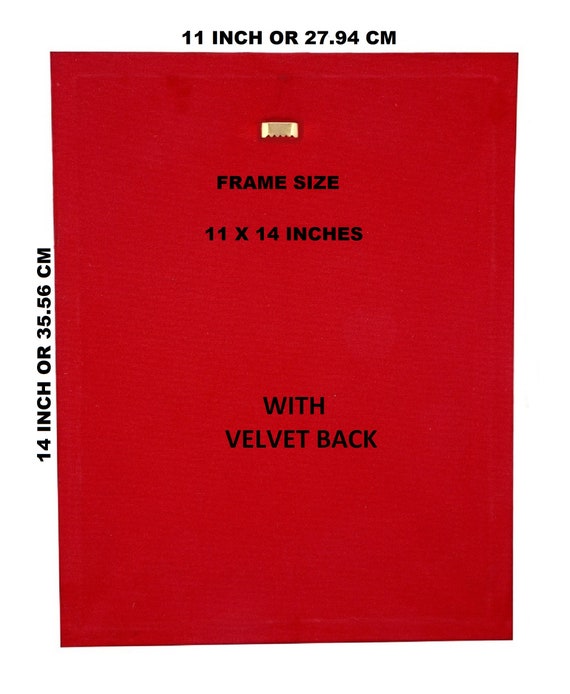This image features a detailed label against a red background, specifying the dimensions and features of a photo frame. At the top, in all capital letters, it reads "11 INCH" or "27.94 CM" horizontally. A small gold metal loop is also visible at the top, likely meant for hanging the frame. The label prominently displays a large rectangle that almost fills the entire space, indicating the frame size. In black text near the middle, it states "FRAME SIZE 11 BY 14 INCHES WITH VELVET BACK." To the left of this text, "14 INCH" or "35.56 CM," the vertical dimension of the frame, is specified. This information suggests that the insert is designed to inform customers of the frame's size, ensuring they select the appropriate frame for their picture, and highlights the velvet backing which prevents the picture from slipping within the frame.